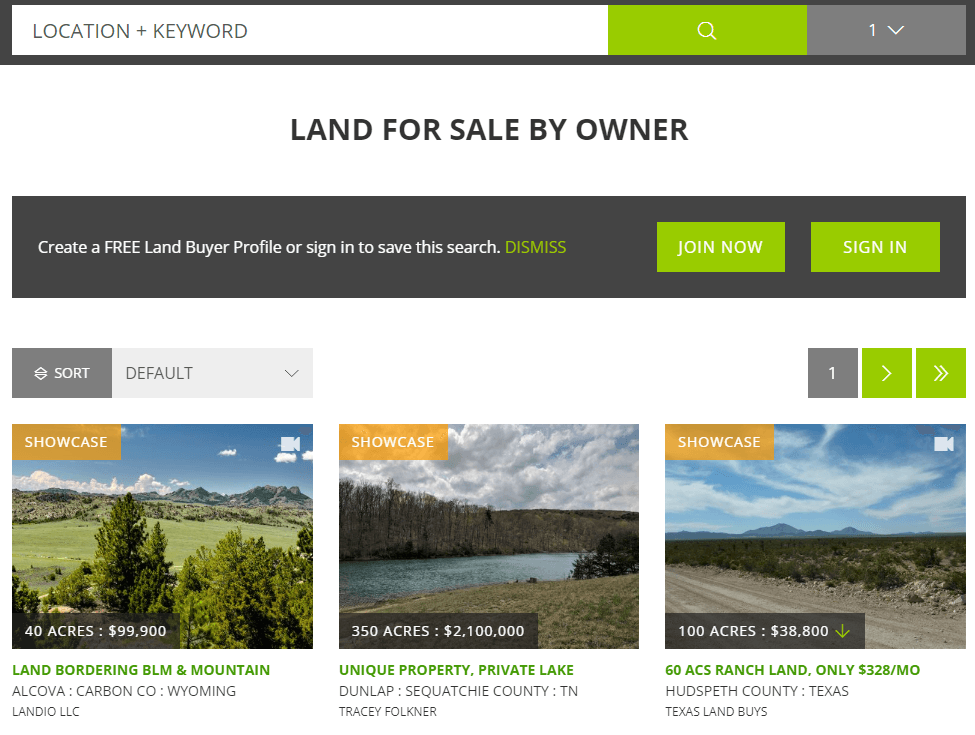The image showcases a search interface for a real estate website, specifically focusing on land for sale by owner. At the top, there is a search bar with placeholders for "Location," a plus symbol, and "Keyword." To the right of the search bar is a long green button featuring a magnifying glass icon, indicating the search function. Adjacent to this is a gray box with the number "1" inside and an arrow pointing downward.

Below the search bar, in bold black text, the heading reads "Land for Sale by Owner." Beneath this is a long gray box containing the text: "Create a FREE land buyer profile or sign in to save this search." To the right of this message is a green "Dismiss" button. Further right, there are two green buttons labeled "Join Now" and "Sign In."

Moving down the page, the layout features three boxes showcasing land listings. The first box displays an image of green mountains, lush trees, and a blue sky. The caption reads "40 acres, $99,900" with additional details in green text: "Land bordering BLM and Milton, Alcova, Carbon Co., Wyoming."

The second box features a large river with trees in the background, labeled "350 acres, $2,100,000." The caption describes the listing as a "Unique property, private lake."

The final box shows an expanse of land with a blue sky and blue mountains, captioned "100 acres, $38,800." Additional details note "60 acres ranch land, only $328 a month, Hudsmith County, Texas."